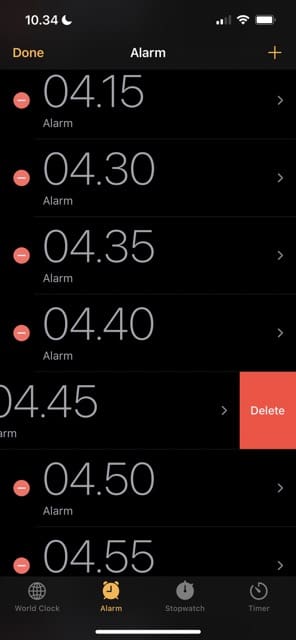A screenshot of a smartphone in night mode displays the details of the alarm settings interface. The entire screen has a dark backdrop indicating night mode. In the upper left corner, the device time reads 10:34 PM, accompanied by a crescent moon icon, signifying Do Not Disturb mode. Two out of four signal bars show, depicting the phone's signal strength, followed by the white Wi-Fi logo, and a white battery icon displaying a sufficient charge level.

Beneath this, in orange text to the left, it says "Done," and in the center, in white text, it states "Alarm." On the right, a gold "+" sign adds options for creating new alarms. Below, the list of alarms are displayed:

1. An alarm set for 04:30 with a red circle featuring a white line through it, indicating that the alarm is active. Below this is the label "Alarm" in gray.
2. Another alarm set for 04:35 follows the same design—red circle with a white line and "Alarm" below.
3. The 04:40 alarm continues this pattern, with the red icon and "Alarm" designation.
4. Similarly, the 04:45 alarm has the identical red circle and white line, but it's sliding left, partially off-screen, revealing a red "Delete" option.
5. The final alarm listed is set for 04:50 and mirrors the same design elements.

The bottom row of icons displays four functionalities:
1. "World Clock" with a globe icon.
2. "Alarm" with an old-fashioned alarm clock icon.
3. "Stopwatch" with a running stopwatch icon.
4. "Timer" with a dial wrapping around the clock icon.

Of particular note is the action on the 04:45 alarm, where the user is in the process of deleting it. The text and time are slightly cut off, with a red box and white "Delete" text sliding in from the right.